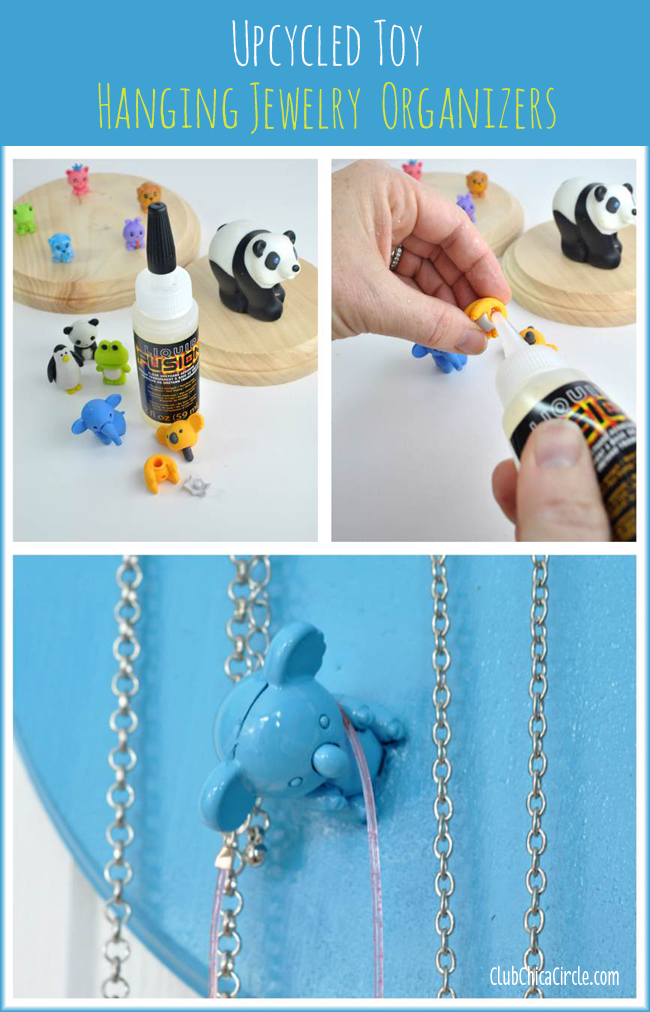A vibrant book cover displays a creative DIY project titled "Upcycled Toy Hanging Jewelry Organizers" in playful white and orange fonts. Set against a blue backdrop, the cover features three descriptive images. The first image highlights a kit with two wooden platforms and an assortment of small, colorful toy animals – including a polar bear, koala, penguin, frog, panda, and a pink elephant. The next image captures the process: a person uses a "Liquid Fusion" glue tube to affix these toys onto one of the wooden platforms. The final image showcases a finished piece – a blue koala firmly glued to a painted podium, repurposed as a whimsical jewelry holder adorned with chains. A noteworthy detail at the bottom reads "clubchicocircle.com", indicating the source of this charming upcycle project.